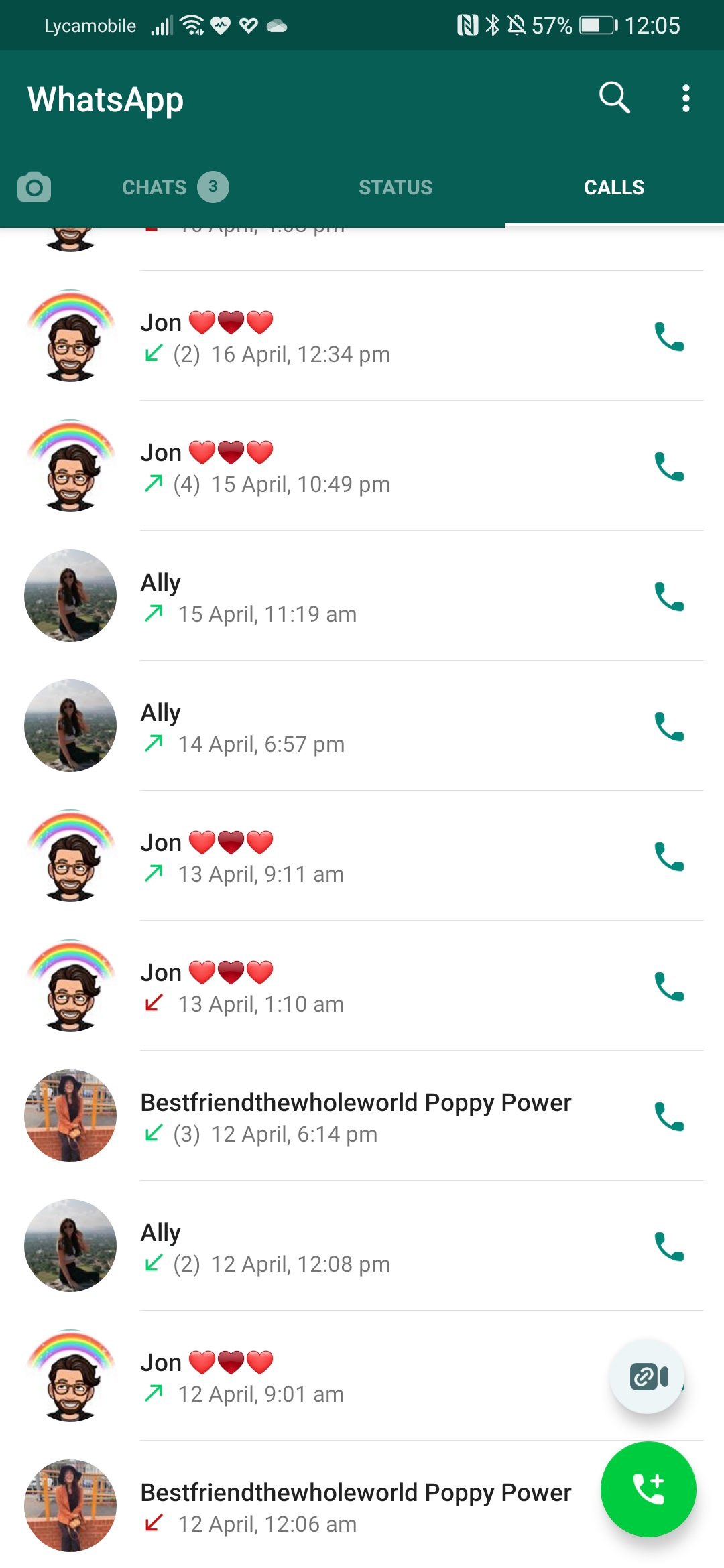The image is a detailed screenshot of a person's WhatsApp call history, taken from an Android phone at 12:05 PM. The top bar of the phone screen reveals the user has a strong cellular connection from Lycamobile and a Wi-Fi connection, showing four signal bars. Additional icons include two heart symbols, a cloud symbol, the NFC icon, and the Bluetooth icon, all active, while the battery stands at 57%. Notable system statuses include the ringtone being off as indicated by a crossed-out bell icon. 

The WhatsApp interface highlights the "Calls" section in white, with tabs at the top for Camera, Chats, Status, and Calls. The Chats tab shows three unread messages. Within the call history, multiple call entries are listed, primarily with contacts named John (depicted with a male emoji with glasses, black goatee, and black hair under a rainbow), Allie (shown with a nondescript female emoji due to the small image size), and a contact named "Best Friend in the Whole World,” also known as Poppy Power, depicted with a female emoji sitting on a bench. Call times range throughout various hours of the day and night, illustrating a pattern of frequent and varied communication.